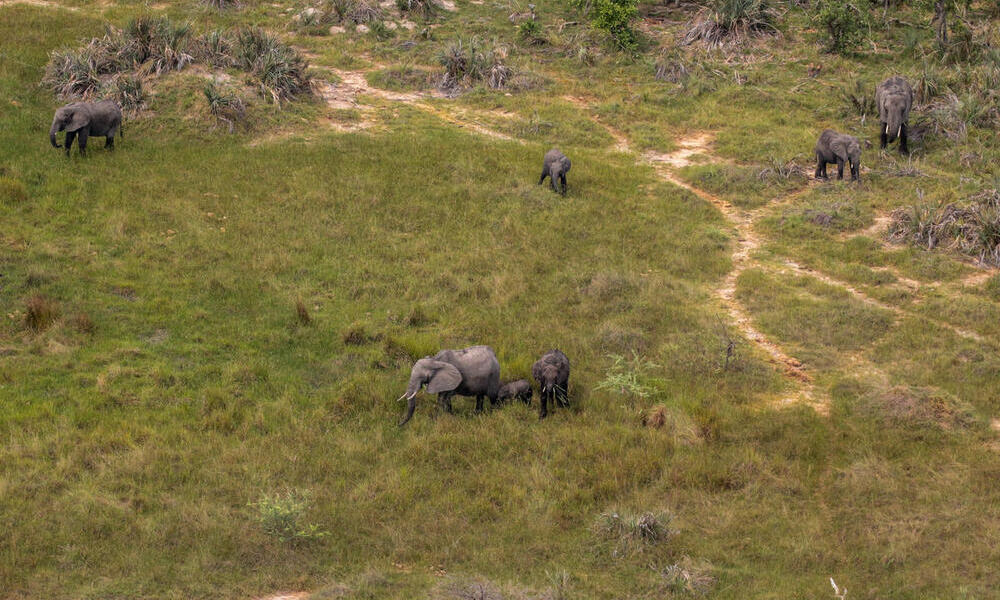The aerial, landscape-oriented image captures a small herd of about seven African elephants scattered across a grassy area. The scene features both lush green and dead grass, with noticeable pathways that have been trampled to form trails. Towards the back of the image, there are taller grasses and some bushes. Prominently in the front and center of the image is a mother elephant with two calves. The herd includes three large adult elephants, two smaller adolescent elephants, and one very young calf. A particularly large adult elephant is located at the top right, standing near a medium-sized adult elephant. The entire composition, captured from a drone, provides a detailed bird's-eye view of these majestic animals in their natural habitat.